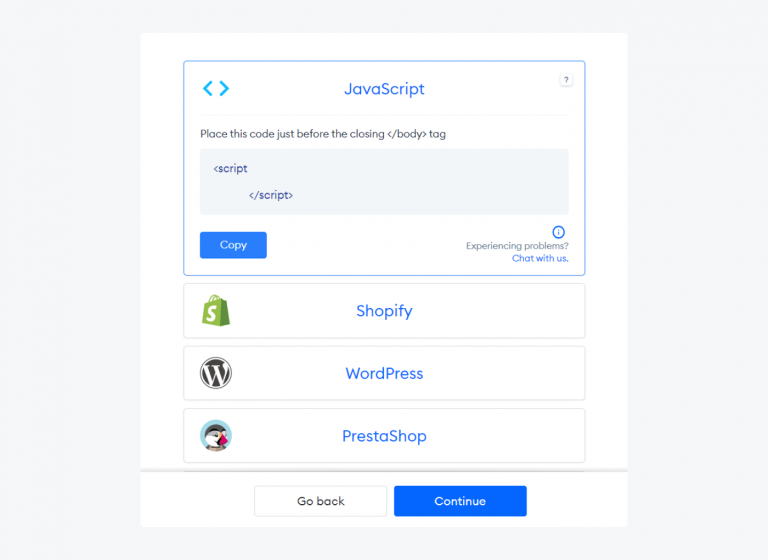This screenshot, taken from a website, features a predominantly off-white to gray background with a central white box. At the top of this box, a squared-off area with a blue underline contains navigation arrows on the top left; one pointing left and the other right. The centered text reads "JavaScript," and on the top right, there is a white circle with a question mark inside.

Directly below this header, there is an instructional text that reads, "Place this code just before the closing </body> tag." Underneath this instruction, a light gray code box displays a snippet starting with "<script>", followed by a blank line, and then "</script>".

Beneath the code box, a blue button labeled "Copy" is present. Adjacent to this button is a blue circle with an eye icon, accompanied by the text "Experiencing problems? Chat with us," where "Chat with us" is a clickable link.

Further down, various platform logos are shown, each within a clickable link. A green shopping bag with an "S," the Shopify logo, is labeled "Shopify." Next to it, a circle with a black background features a "W" and is labeled "WordPress." Following is a blue circle displaying a colorful bird icon labeled "PrestaShop."

At the very bottom of the image are two buttons: a neutral-colored "Go Back" button and a blue "Continue" button, indicating the latter is the likely choice for advancing.